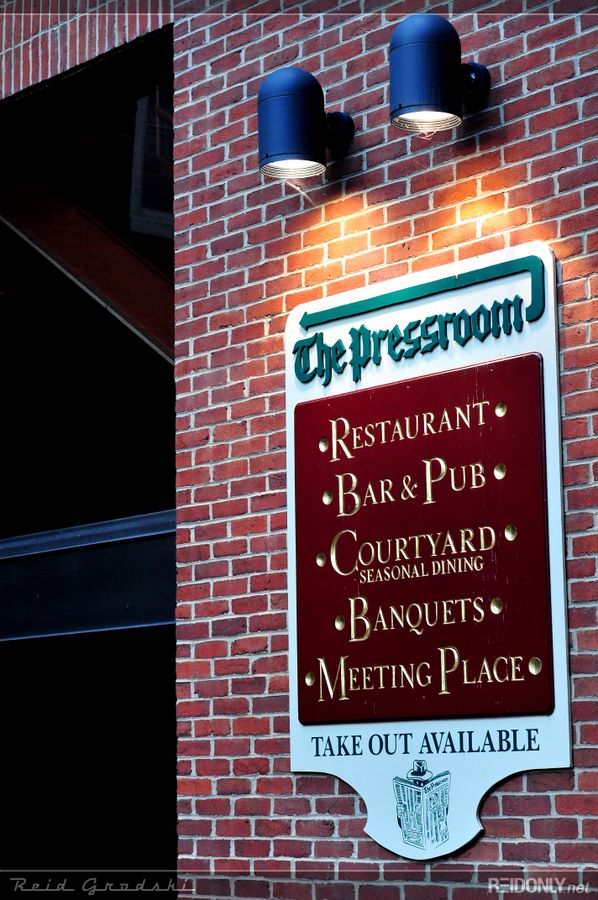The image showcases the side of a red brick building, dominated by a large brick wall that occupies the entire right side and extends to the top of the frame. Centrally positioned, though slightly off to the right, is a prominent sign under two black cylindrical lights. The sign reads: "The Press Room" with directional details pointing to the left. The text on the sign is divided among different colored sections: "Restaurant, Bar & Pub, Courtyard, Seasonal Dining, Banquets, Meeting Place" written in green text on a red background, and "Takeout Available" in white text on the white part of the sign. There is also an image of a man reading a newspaper. The setting appears to be outside a restaurant, possibly at night, as suggested by the dark tones around an opening on the left side which remains indistinct. The colors present in the image include black, brown, white, green, red, yellow, and tan. Additionally, a watermark reading "Read Gray Grad Ski" is on the bottom left, and "Read Only Dot Net" is found on the bottom right.